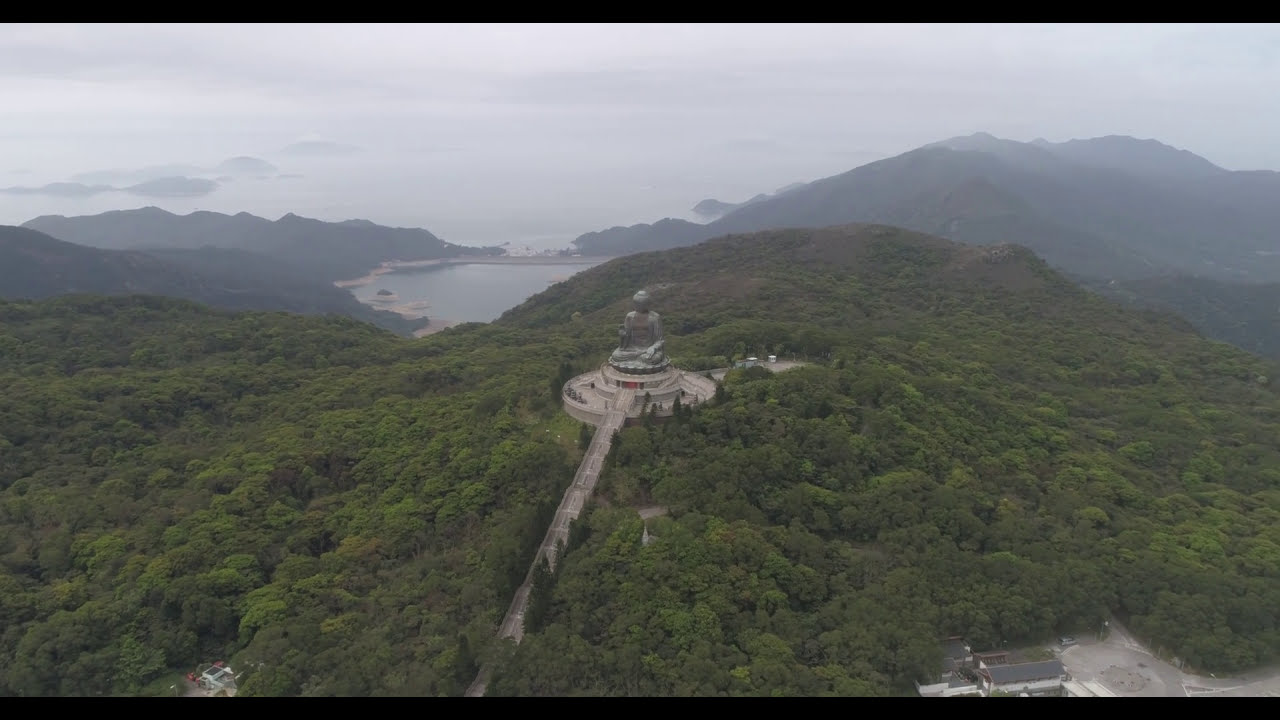The image captures a giant Buddha statue situated at the heart of a forested area rich with trees and greenery. The Buddha statue, several hundred feet tall and seated in a lotus position, dominates a round concrete courtyard surrounded by a complex of buildings. Narrow stairs extend from the courtyard, leading to this circular area where people are seen milling about. In the background, hazy gray clouds shroud distant mountains and a small lake or bay. The overall setting suggests a serene natural environment, possibly in South America, with the statue serving as a significant focal point amidst the lush landscape.